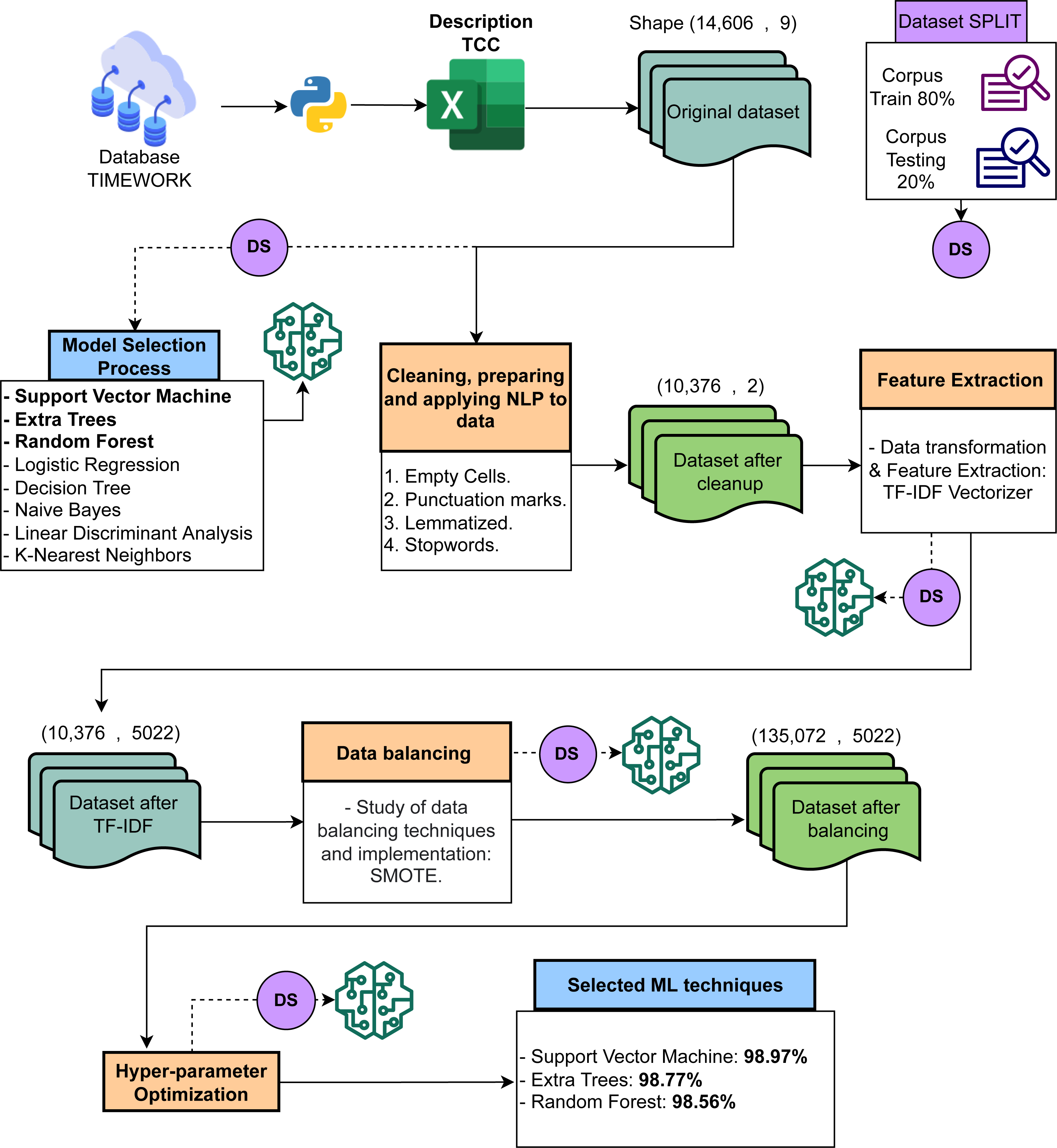This detailed flowchart against a white background meticulously outlines the various stages of data analysis, splitting into multiple interconnected paths. Starting at the upper left, a blue cloud labeled "database time work" branches off to show the initial data input method. This flows into several key stages, depicted through distinctive icons and color-coded sections such as blue, yellow, green, pink, and purple for easy visual differentiation.

The flow moves right to a section with a yellow and blue icon, then proceeds to an icon showing an Excel document titled "description TCC." Following this, it transitions to a stage labeled "Shape 14,606,9," featuring an icon marked “original data sheet.”

Diving deeper into the data preprocessing steps, there is a detailed breakdown under the label "cleaning, preparing, and applying NLP to data." This includes explicit steps for handling empty cells, punctuation marks, lemmatization, and removing stop words. Their interconnected flow is indicated by solid and dotted lines showing conditional and sequential progressions.

As the chart continues, it moves downward and meanders horizontally, eventually dotting through crucial phases such as "hyperparameter optimization." This leads you to a prominent section in purple labeled "dataset split," paralleling the model training stages.

In the final stretch, it converges at a bottom box labeled "selected ML techniques." This section details performance metrics for various machine learning models: Support Vector Machine (98.97%), Extra Trees (98.77%), and Random Forest (98.56%). Throughout, the layout includes arrows and images such as a brain-shaped circuit board, which symbolize the complex processes and technological tools in use.

Overall, this comprehensive diagram dynamically illustrates each critical step from data handling to machine learning model selection, emphasizing both the complexity and methodical approach of the data analysis workflow.